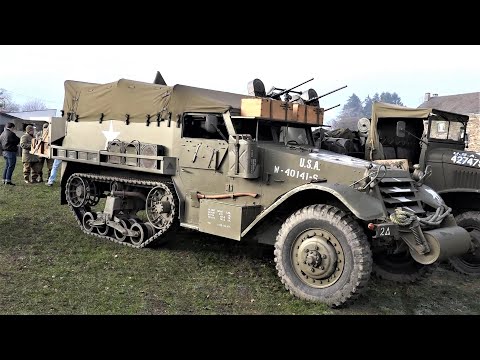In this photograph, a military tank, painted in army green, prominently features a white star symbol and the marking "USA M-40141-S" on its side. The tank's mounted guns are clearly visible. Behind the tank, four individuals stand, two of whom are wearing blue jeans, hats, and coats. Beside the tank, an army jeep also marked with "USA" and the serial number "42747" can be seen. The scene is set outdoors on a grassy area, under a cloudy sky. In the background, a stone building and several trees are visible, adding context to the setting.